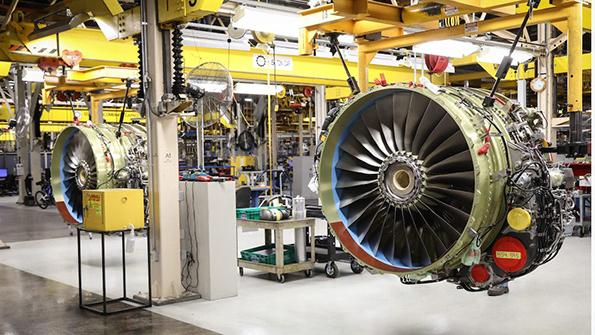The image shows the interior of a large, well-lit manufacturing plant designed for high-tech industrial work. Dominating the scene are two enormous jet engines suspended from sturdy, yellow-painted steel I-beams. These engines consist of large, cylindrical metal frames housing central fan blades. Surrounding these cylinders are a network of valves, pipes, and multiple mechanical components, including two diagonally positioned pistons on each engine. The engines also feature several red and yellow cylindrical components. The floor is white and gray, dotted with various industrial tools and rolling carts holding equipment. The backdrop of the room includes more industrial tools and gauges, contributing to the plant's technical atmosphere. The ceiling is supported by multiple metal pillars, and cranes are also visible, hinting at the heavy-duty nature of the machinery produced and assembled in the facility.